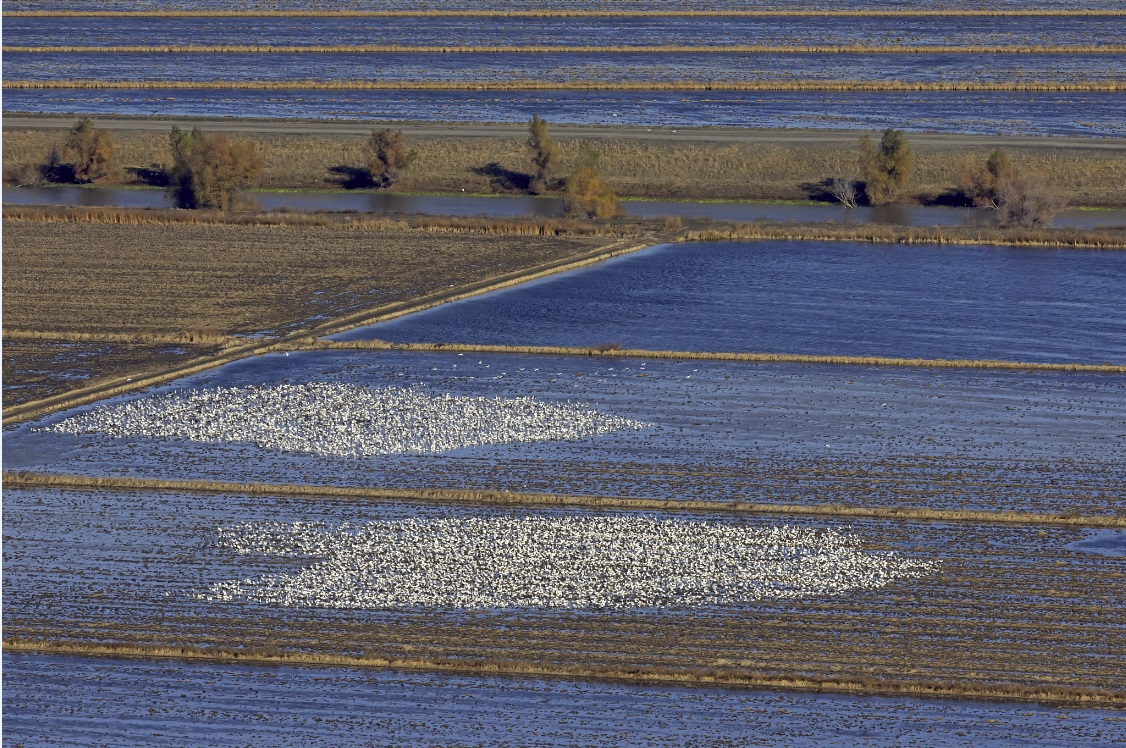The photograph captures a bird's-eye view of irrigated rice fields in California, showcasing a complex agricultural landscape segmented into various sections by levees and waterways. The foreground reveals four submerged sections, with the mid-sections prominently featuring dense clusters of white waterfowl, likely geese, resting in the shallow waters. The upper portion of the image transitions into fallow, brownish-green grasslands interspersed with green shrubs. These grasslands flank a series of tiered irrigation fields, each bound by levees to manage the water levels. The image, potentially taken from a drone or elevated structure, highlights two primary fields divided by a central waterway, adjacent to which lie the dense congregations of white birds, appearing as bright patches against the muted tones of water and crop.